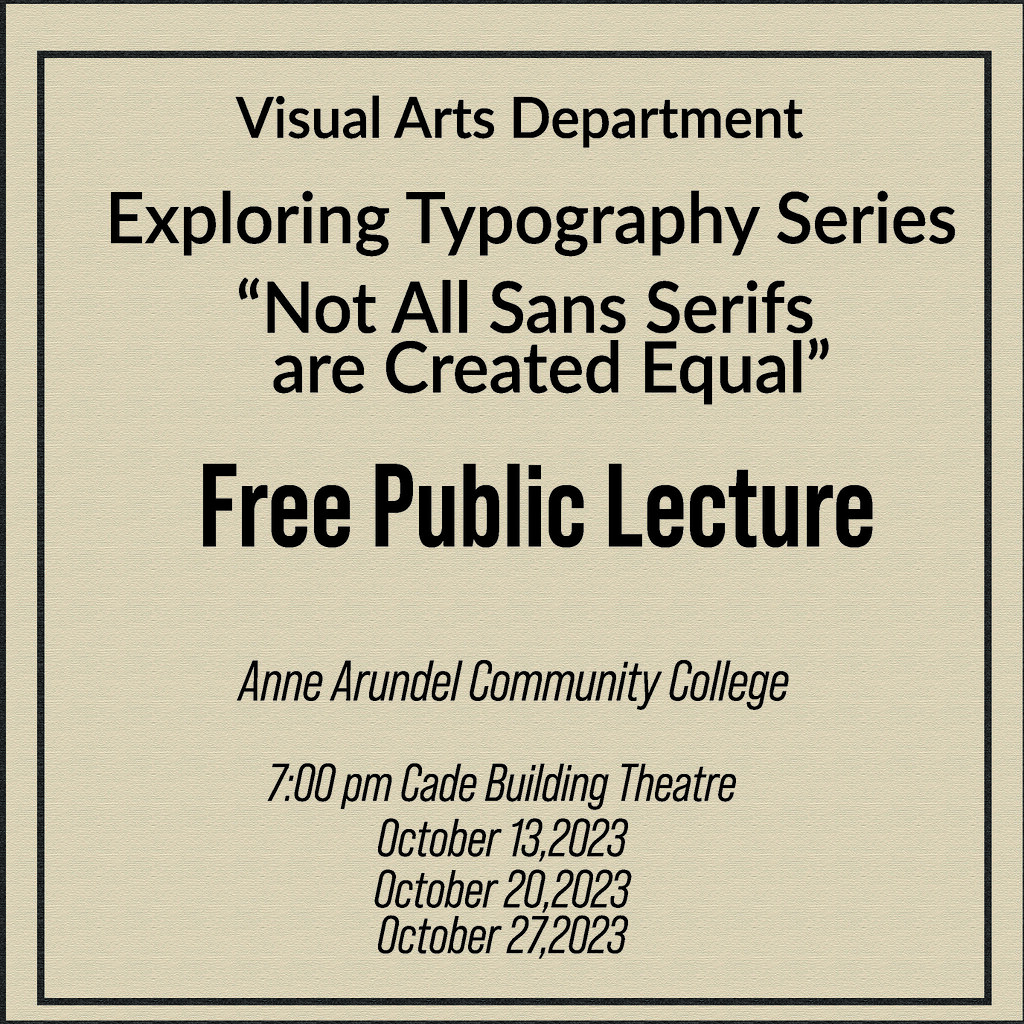This is an advertisement for a free public lecture, set against a light tan background with all text in black. At the top, it reads "Visual Arts Department" followed by "Exploring Typography Series." The quote "Not all sans serifs are created equal" is prominently displayed beneath the series title. Centrally positioned in bold black letters are the words "Free Public Lecture." Below in smaller, almost grayish text, it details "Anne Arundel Community College," followed by the location "7 p.m. Cade Building Theater." The dates of the lecture are listed consecutively: "October 13, 2023," "October 20, 2023," and "October 27, 2023."